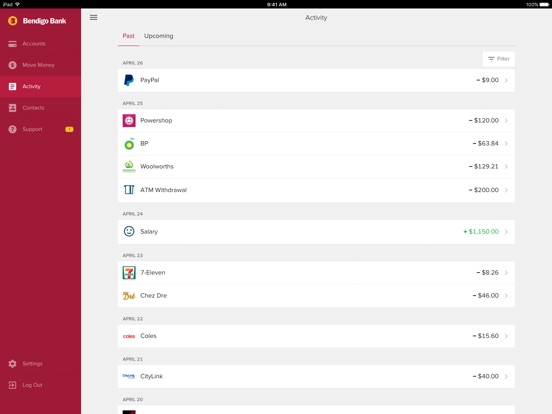A screenshot of a PayPal account summary is shown against a slightly blurry background resembling Bendigo bark. The top part of the screen, displaying the iPad status, reads "9:51 a.m." with a full battery at 100%. Below, various account sections, such as "Move Money," "Activity," "Contact Support," "Settings," and "Log Out," are visible. The "Activity" tab highlights several transactions dated from April 20th to April 26th. On April 26th, there is a negative PayPal transaction of $9. Transactions on April 25th include a power shop payment of $120, a BP charge of $63.84, a Woolworths expense of $129.21, and an ATM withdrawal of $200. A salary deposit of $1150 is listed without a date. Additional transactions include a 7-Eleven purchase of $8.26, a Shez Dre transaction of $46, a Coles expense of $15.60, and a City Link charge of $40, all dated April 20th.